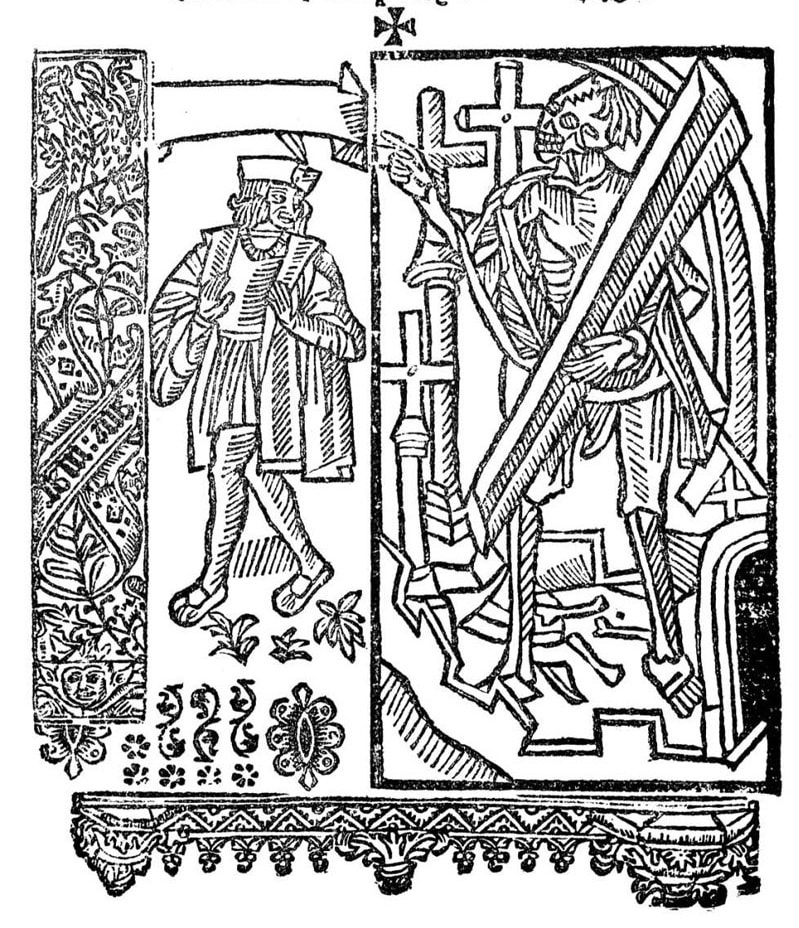This black and white wood print or engraving, likely from the 16th or 17th century, is divided into two sections and features two prominent figures. At the top center, there's a symbol associated with the Knights Templar. 

In the left pane, a man, dressed in ancient attire including a cloak, hat, necklace, and sandals, stands with his hands raised as if about to clap. He has an expressive look, glancing over his left shoulder towards the right pane. Surrounding him are detailed illustrations of flowers and swords.

The right pane presents a more ominous scene dominated by a skeletal figure dressed similarly to the man in the left pane, complete with ancient clothing but starkly in skeletal form. This skeleton, holding a long beam-like object, stands among crosses and small pillars adorned with crucifixes, with bones scattered at its feet. There is a noticeable archway behind the skeleton, enhancing the scene's antique ambiance. The juxtaposition of life and death is striking, especially with the skeletal figure pointing ominously across the way. The delicate engraving details and symbolism throughout the work suggest an age-old commentary, rich with historical and visual intricacies.